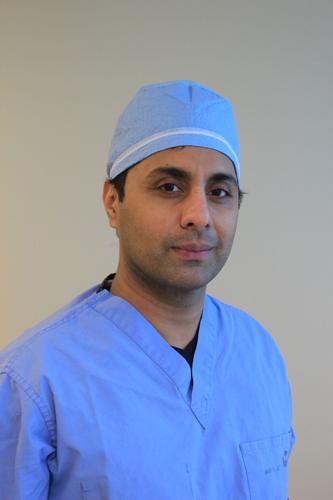The image is a small vertically-oriented photograph depicting a doctor in what appears to be a professional setting. The background is a muted gray, directing focus onto the doctor, who is dressed in light blue scrubs and a matching scrub cap adorned with a white band at the bottom. He also wears a dark undershirt beneath his scrub top, which features some unidentifiable lettering on the pocket located on the left side of his chest. The doctor has a dark complexion and short black hair, mostly concealed by the scrub cap, with a little bit peeking out. His face is defined by a stubble beard and mustache. He is wearing glasses and gazes at the camera with an intent expression, suggesting he might be about to perform surgery or explain a medical procedure. The photograph captures him from the chest up, leaving his arms out of the frame, and presents him in a slightly quarter-side profile starting from the left.